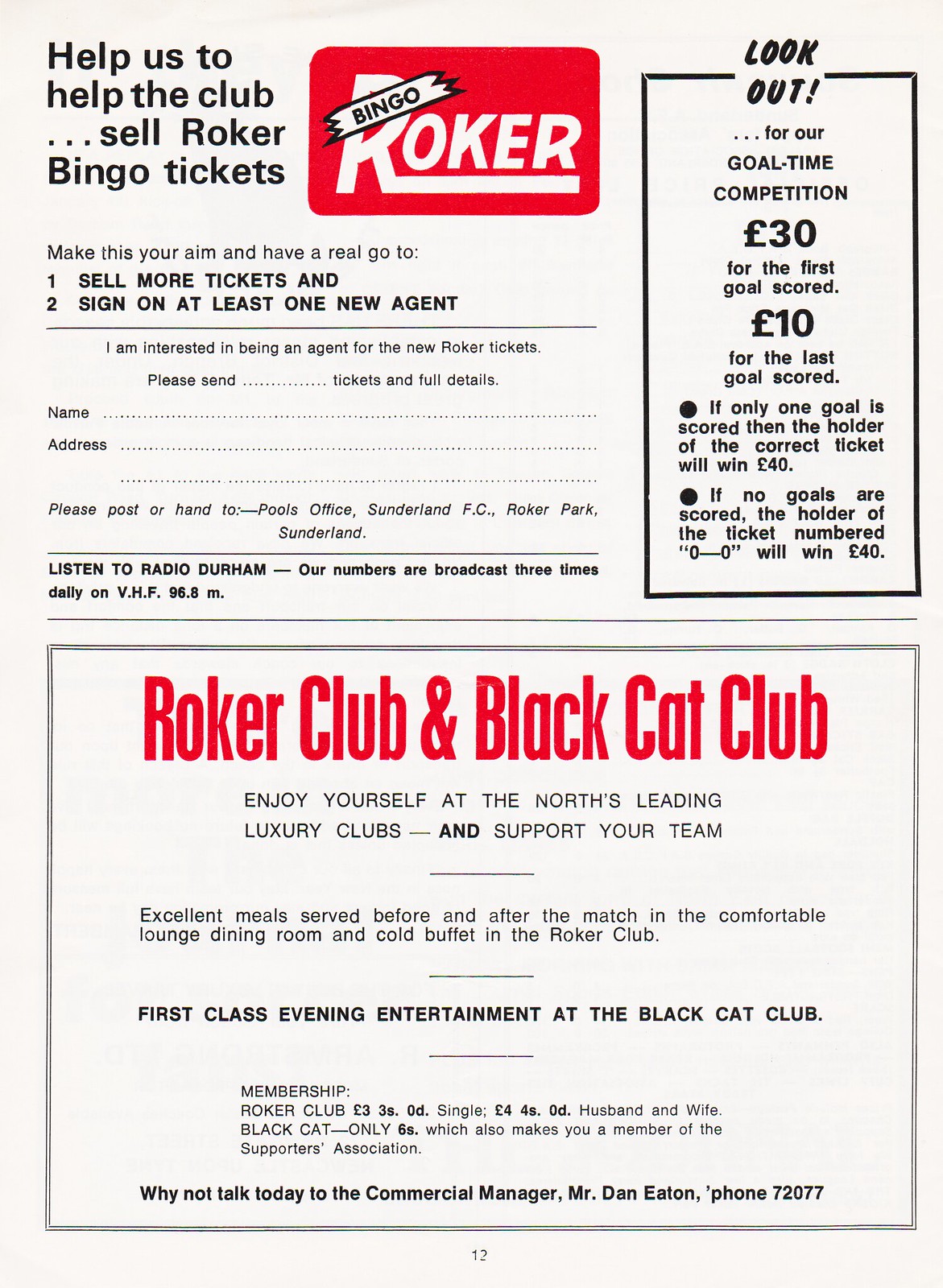This tall, rectangular poster has a primarily off-white beige background and promotes the sale of Roker bingo tickets. In the top left corner, black text reads, "Help us to help the club... sell Roker bingo tickets." Beside this text, a red, rounded rectangle features the logo "Bingo Roker" in large white letters, with a diagonal slash beneath the 'R' and 'O'. Below this is an order form where individuals can fill in their name and address and select the number of tickets they want.

On the right side of the poster, a vertical rectangle highlights the "goal time competition," offering £30 for the first goal scored and £10 for the second goal scored, with specific conditions for prize allocations if fewer goals are scored.

Further down, a large red rectangle displays the names "Roker Club" and "Black Cat Club" in bold red letters. Below this, smaller black text invites people to "Enjoy yourself at the North's leading luxury clubs and support your team." The advertisement also mentions the availability of first-class evening entertainment and provides contact information for Mr. Dan Eaton, the commercial manager, encouraging individuals to get in touch.